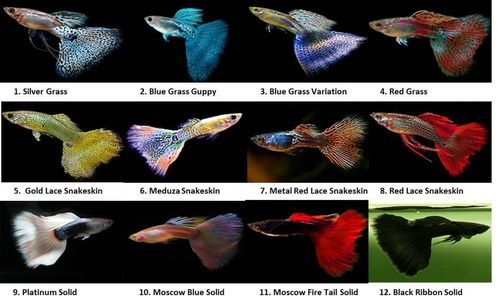The image is a detailed, colored chart showcasing 12 distinct types of betta fish, each identified by name and arranged in a three-by-four grid on a predominantly black background, except for the last fish which has a greenish background. Starting from the top left, number 1 is Silver Grass, a vibrant fish with a red body and a striking white and blue tail. Number 2 is Blue Grass Guppy, featuring a silver body and a vivid blue tail. Number 3, Blue Grass Variation, presents a yellow body with a purple tail. Positioned in the upper right corner, number 4 is Red Grass, predominantly red with hints of blue spots. Below Silver Grass, in the middle of the second row, number 5 is Gold Lace Snakeskin, notable for its golden hue. To its right, number 6 is Medusa Snakeskin, an intriguing mix of oranges, purples, and yellows. Number 7 is Metal Red Lace Snakeskin, showcasing a bronzish color with blue tinges. Number 8, Red Lace Snakeskin, features red accents with a bronze-toned body. In the bottom left of the grid, number 9 is Platinum Solid, with a striking white-silver tail and a darker body. To the right of Platinum Solid, number 10 is Moscow Blue Solid, reddish with blue tinges in the tail. Number 11, Moscow Fire Tail Solid, has a black body contrasted by a bright, dark red tail. Finally, in the bottom right corner, number 12 is Black Ribbon Solid, showing a silhouette on a greenish-black background. Each fish is uniquely colorful, ranging from shades of yellow, blue, and red to white and bronze, making the chart a vivid and informative representation of betta fish varieties.